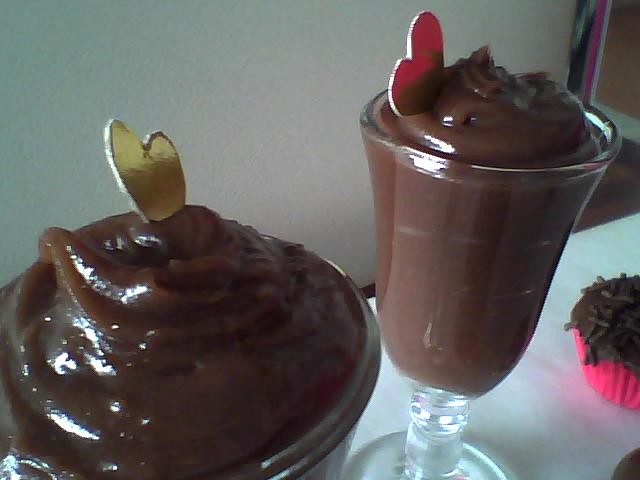This close-up image showcases three delectable desserts arranged on a pristine white countertop against a light-colored wall background. On the far right, there is a chocolate cupcake adorned with chocolate sprinkles, partially encased in a pink wrapper. To the left of the cupcake, there are two cocktail glasses, elegant with short stems and bell-shaped bowls. Each glass contains what appears to be rich, dark chocolate mousse. The mousse in the glass on the right is decorated with a red candy heart, while the mousse in the glass on the left features a golden heart. The meticulous detailing of the desserts and their vivid contrasts elevate the visual appeal of the image, creating a delightful feast for the eyes.